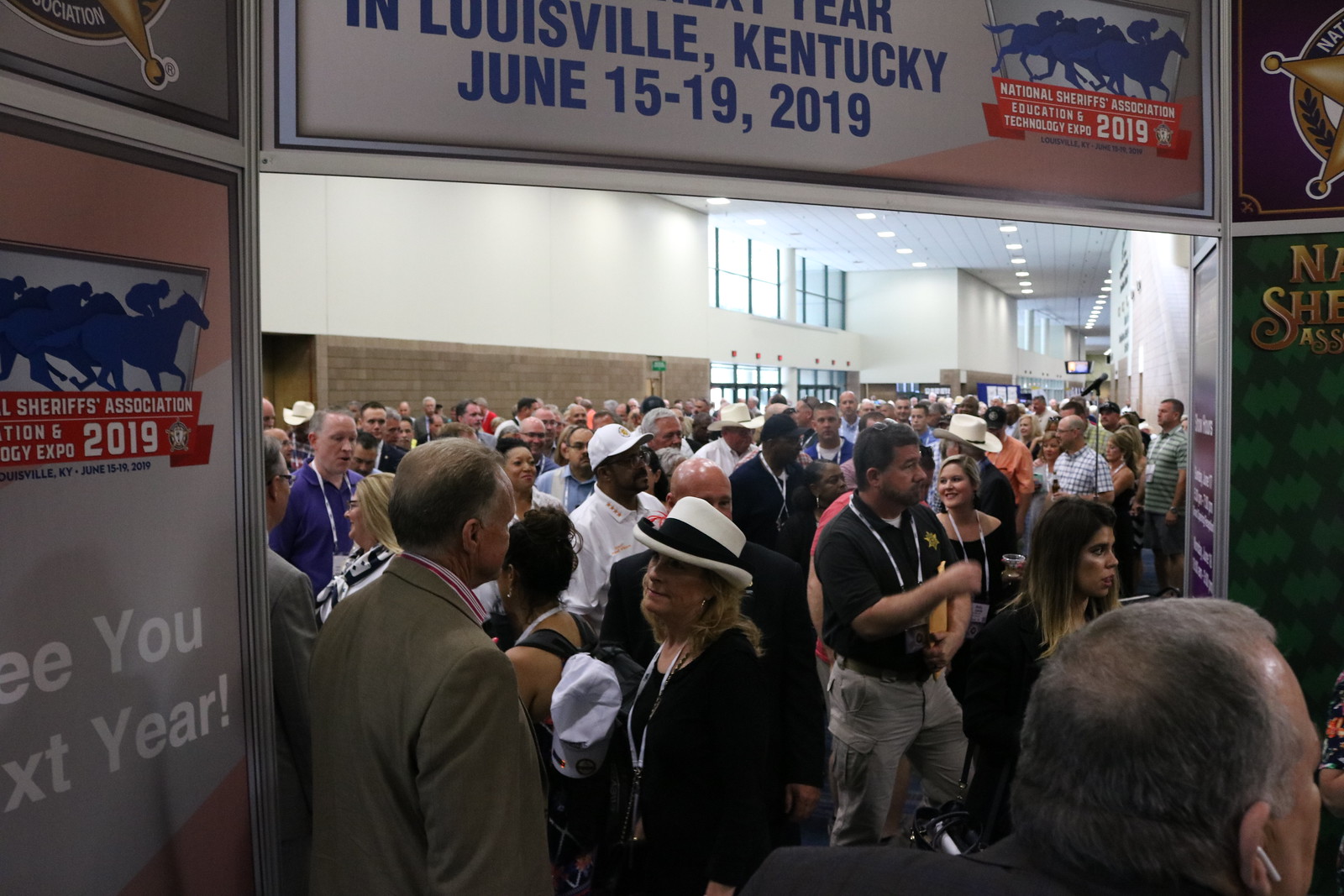The photograph depicts a bustling indoor setting, likely a convention center or Expo Hall, crowded with nearly a hundred individuals. The central focus is an open doorway leading into a long hallway teeming with attendees. Above the doorway, prominent banners announce the "National Sheriffs Association Education and Technology Expo" held in Louisville, Kentucky, from June 15 to 19, 2019.

The crowd appears to be largely composed of individuals associated with the sheriffs' profession, as indicated by the star badges adorning their clothing and hats. Numerous attendees wear lanyards, likely for identification purposes. The attendees are dressed casually, with many in black shirts, and a few in white or other colors. Both men and women are present, engaging in conversations and activities.

In the image's background, additional doorways lead to the building's exit, suggesting it's daytime outside. The top of the image features some windows and ceiling lights, adding to the indoor ambiance. A distinctive logo of a blue horse with riders, suggesting a sheriff's theme, appears in the top right.

The bottom-right corner shows the back of a person with short gray hair and an AirPod in their ear, adding a personal touch to the busy scene. Additional signs in the hall, such as "see you next year," enhance the sense of a large, organized event, complete with various decorative elements in blue, white, and red.